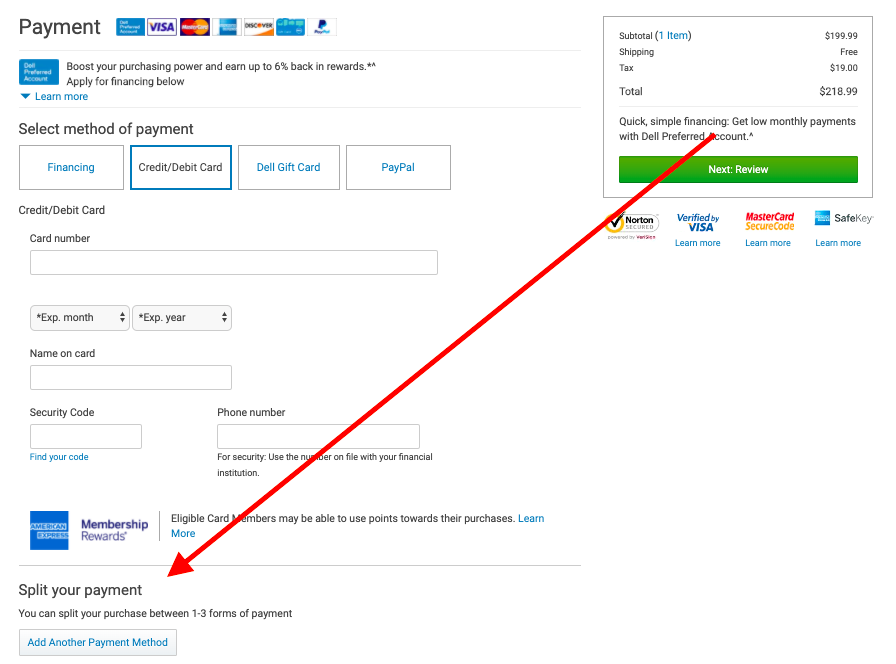This is a detailed screenshot of a payment screen. At the top left, the word "Payment" is prominently displayed in black. Below this, various payment options are listed: "Debit Preferred Account," followed by the icons for Visa, MasterCard, American Express, Discover, an unknown symbol, and PayPal.

Under these options, there's a message encouraging users to "Boost your purchasing power and earn up to 6% back in rewards." It also prompts users to "Apply for financing below," with a blue "Learn More" link accompanied by an arrow. 

Further down, the section "Select Payment Method" provides four choices: Financing, Credit/Debit Card, Deli Gift Card, and PayPal. Below that, under "Credit/Debit Card," several fields are available: a box for the card number, a drop-down menu for the expiration month with up-and-down arrows, another drop-down for the expiration year, a box for the name on the card, and a box for the security code, which includes a blue "Find Your Code" link. There is also a box for the phone number, accompanied by a note advising to "Use the number on file with your financial institution."

An American Express logo appears underneath, with a message about "Membership Rewards" explaining that eligible card members may use points towards their purchases, along with a "Learn More" link. Below this, the option to "Split your payment" is presented, allowing users to divide their purchase between one to three forms of payment, and a prompt to "Add another payment method."

To the right at the top, the payment breakdown is summarized: "Subtotal (1 item): $199.99," "Shipping: Free," "Tax: $19," leading to a "Total: $218." A message about "Quick, Simple Financing" offers "Low monthly payments and Deli Preferred Account" next to a green "Review" button.

At the bottom of the screen, security logos for Norton Antivirus, Verified Visa, MasterCard SecureCode, and American Express SafeKey are displayed. Additionally, a red arrow points from this box to the "Split your payment" section on the other side of the screen.